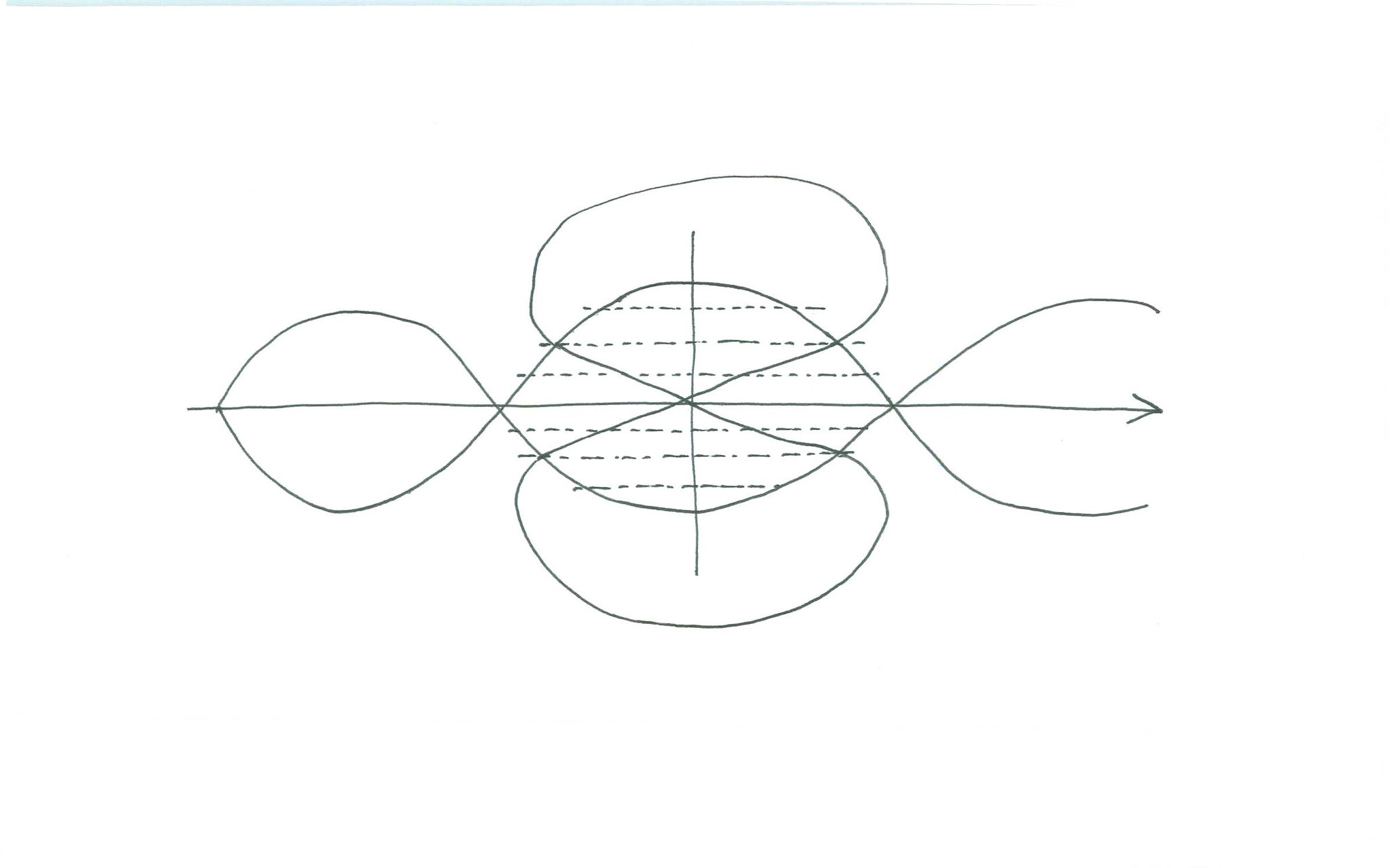This image features a complex composition of various lines and shapes, rendered in shades of black and white. The central focus is a horizontal line oriented from right to left, culminating in an arrow pointing to the left. Surrounding this horizontal line is a helical structure, composed of two intertwining lines. The helix terminates near the left arrow, leaving the endpoint open. Additionally, the middle segment of the helix is intersected by dotted horizontal lines extending downward.

Bisecting the entire composition is a vertical line that cuts through the central area. Encircling this vertical line is another helix, which forms a figure-eight pattern. The crossover point of this figure-eight is slightly off-center, giving the impression of a hand-drawn line with no perfectly straight edges. The image has a sketch-like quality, with all lines appearing slightly gray and imperfect, contributing to a freeform, artistic aesthetic.